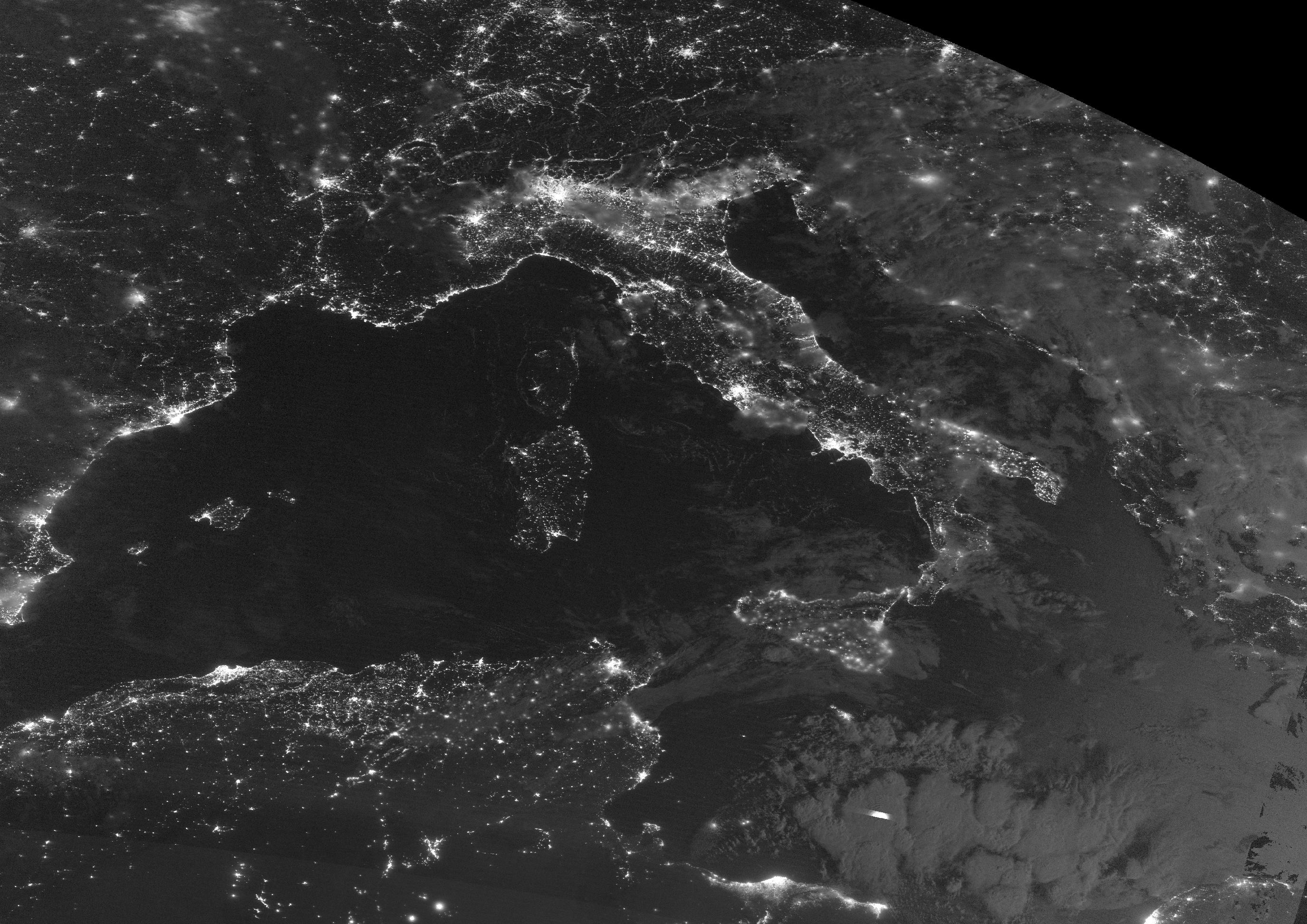This image appears to be a satellite or computer-generated representation of Earth, focusing on Italy. Dominating the center of the scene, Italy is distinctly outlined in a boot-like shape with Sicily clearly visible at the bottom. The overall view is in black and white, with the land areas illustrated by numerous white, sparkly dots, likely representing city lights, indicating heavily populated regions. Major cities are prominently illuminated, while the surrounding water is rendered in solid black, devoid of any lights. The darkness extends mostly around the image, suggesting the vastness of space. Towards the bottom, hints of additional landmasses are visible but less illuminated compared to Italy, signifying fewer urban centers. Notably, the upper right corner shows an all-black expanse, possibly the vastness of space, while a faint arc might suggest the curvature of the Earth. To sum up, Italy is brightly lit, standing out against the dark backdrop, with clearly visible shorelines and hints of the surrounding geographical features.